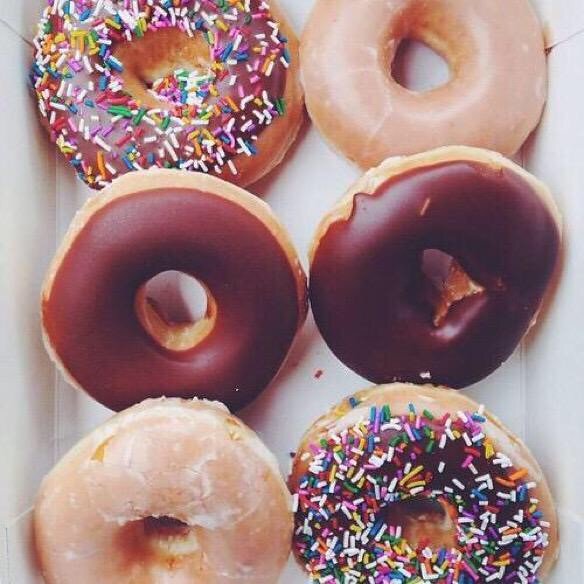An indoor, close-up color photograph captures a white box containing six fresh, untouched doughnuts organized in two vertical columns of three each. The doughnuts are evenly spaced with their round holes clearly visible. The top left doughnut features chocolate icing with a mixture of white and multicolored elongated sprinkles. To its right, the doughnut is simply glazed with a rich, translucent whitish coating, pristine and smooth. The central row showcases two identical doughnuts with a chocolaty glaze, while the doughnut at the bottom left corner has the same glazed appearance but shows slight signs of icing chipping off, indicating its freshness. Finally, the bottom right doughnut mirrors the top-left one with chocolate icing and multicolored sprinkles. The box flaps are visible, and there are no shadows, suggesting the photograph was taken under bright, overhead lighting, accentuating the inviting texture and details of the doughnuts.